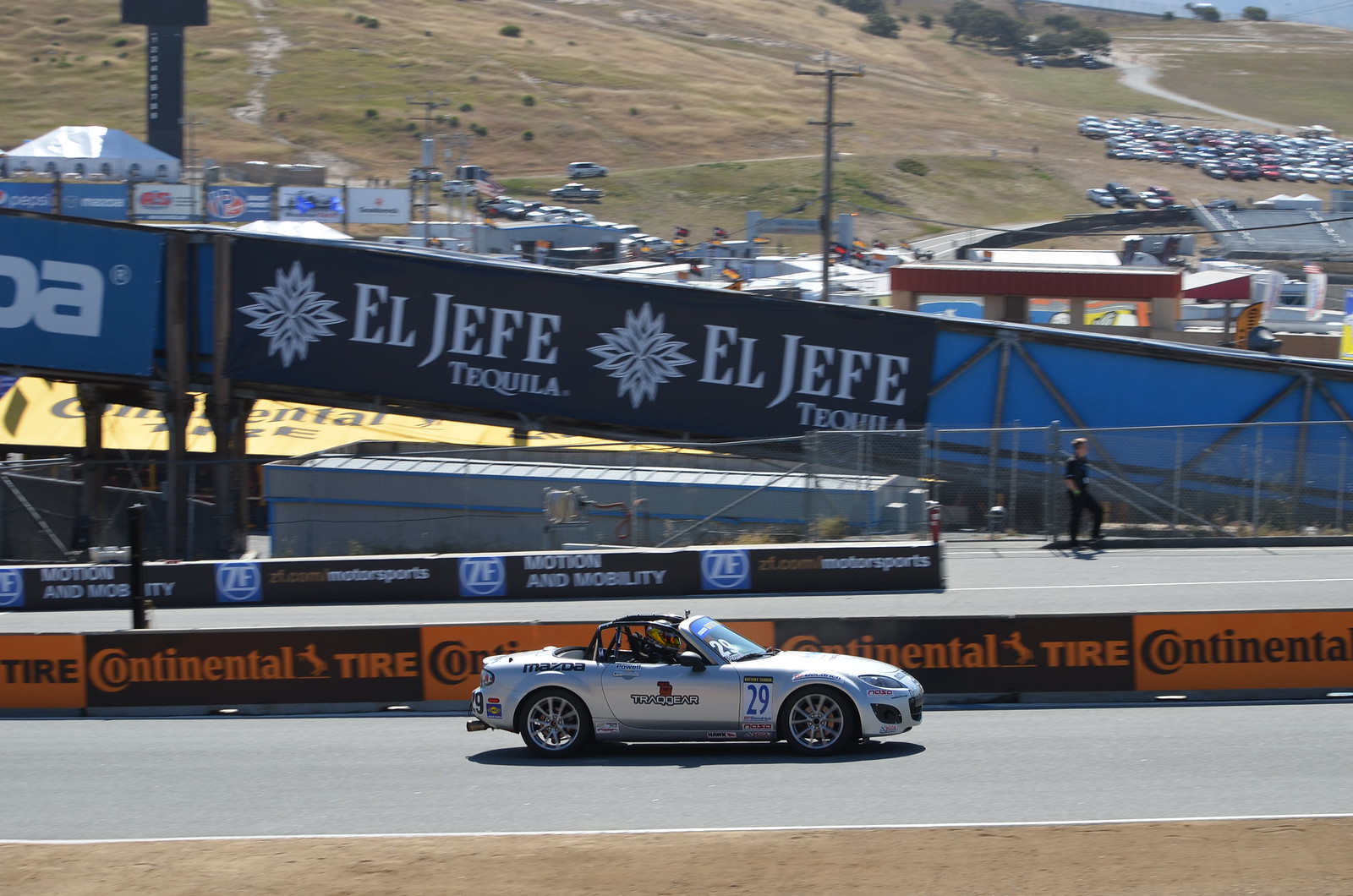The photograph captures an outdoor racetrack scene featuring a gray, two-door Mazda sports car, adorned with numerous stickers and marked with the number 29. The vehicle, which is a one-seater convertible equipped with a roll cage and driven by a helmeted driver, is moving left to right on the gray track. Prominent advertising along the edge of the track includes an orange and black Continental Tires logo, as well as banners for ZF.com Motorsports and motion and mobility. A man walks along the fence line. The background reveals a grassy hill dotted with parked cars and various buildings. The scenic vista also includes distant roadways, additional vehicles scattered across a valley, and a black sign mounted high on a white building. The photograph is wide and rectangular, capturing not only the car and its immediate surroundings but also the broader landscape of the racetrack environment.